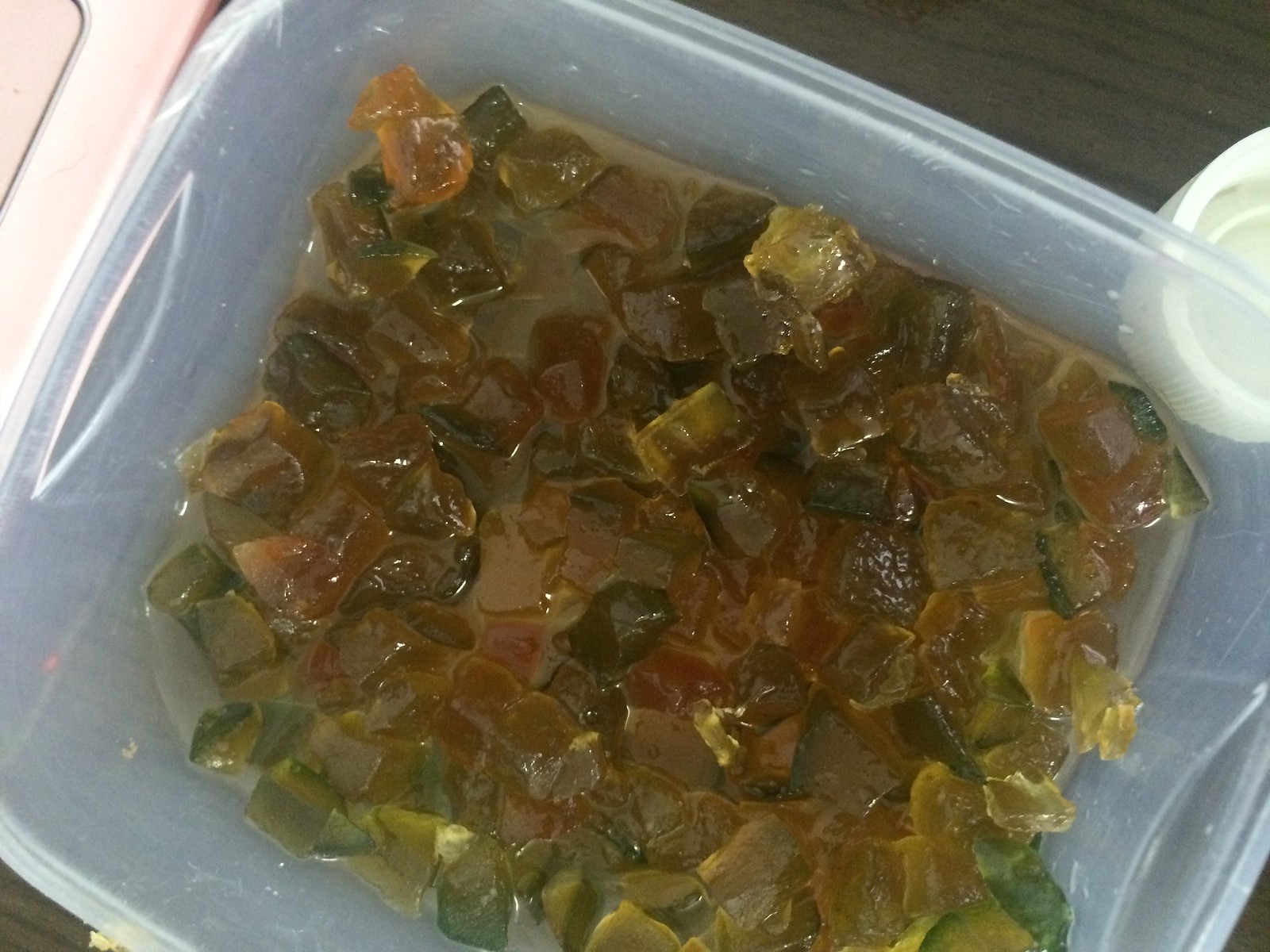In the image, there is a clear, large Tupperware container filled with a gelatinous, sticky mixture of green, yellow, and orange gummies, giving it a fruit salad appearance. The Tupperware container is positioned on a brownish wood table, possibly a picnic table, and the lid is partially attached, sitting to the left. To the right of the Tupperware, there is a white cup or mug. The contents inside the Tupperware are varied with dark, light, and yellow bits immersed in a liquid, enhancing the impression of a colorful, possibly pickled relish or a gum-based fruit jelly mix.